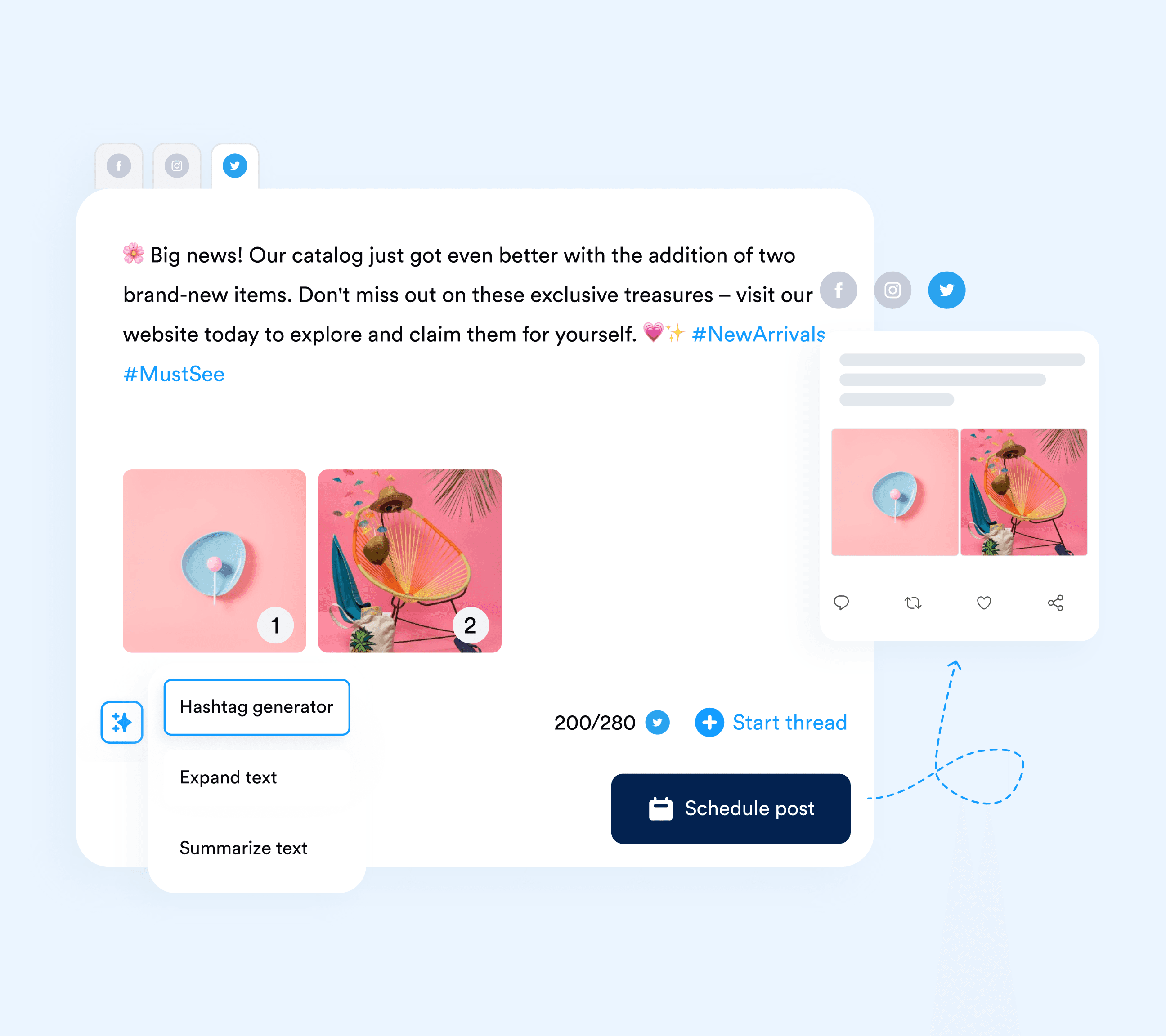The image is a detailed screenshot depicting the interface of a social media management app. The entire background of the image is a light blue, creating a cohesive and visually appealing backdrop. 

On the left side of the square, there are three social media icons: Facebook, Instagram, and a highlighted Twitter icon, indicating the active social media platform. Beneath the Twitter icon, there's a significant white text box containing the caption written for a Twitter post. It reads: "Big news! Our catalog just got even better with the addition of two brand new items. Don't miss out on these exclusive treasures. Visit our website today to explore and claim them for yourself. #NewArrivals #MustSee."

Below this text box, there are two smaller images labeled "1" and "2," likely representing visual content meant to accompany the Twitter post.

Further below, three buttons are displayed: "Hashtag Generator," "Expand Text," and "Summarize Text." The "Hashtag Generator" button is emphasized with a blue rectangle outline, signifying its current selection.

To the right, a counter shows "200 out of 280 tweets," indicating the character count for the post. Adjacent to this, there’s an option to start a thread with a "+ Start Thread" button, and a "Schedule Post" button for timing the post's release.

Lastly, an arrow icon emerges, suggesting the capability to seamlessly post or manage the content across social media platforms. The overall impression is that the app facilitates the creation, hashtag optimization, and scheduling of posts for Facebook, Twitter, and Instagram.